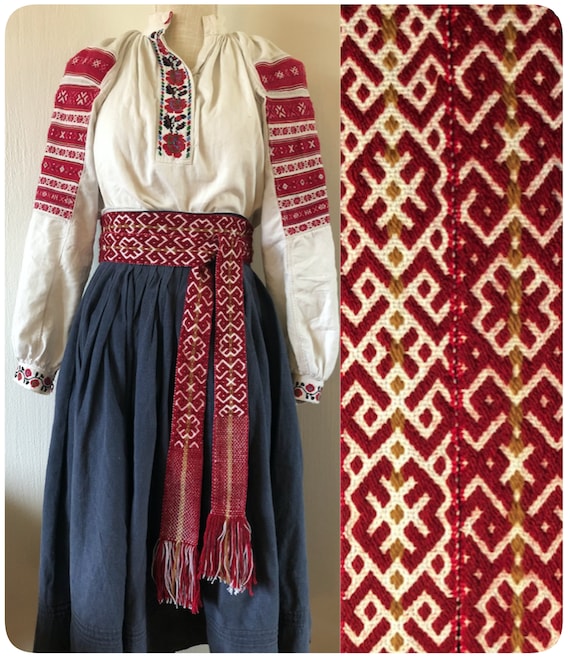The image on the left showcases a vintage-style dress, featuring a distinctive red and white belt at its center. The belt, adorned with intricate X and diamond-like patterns, appears handmade and adds a clock-like charm to the attire. The lower part of the dress is a deep blue-gray, contrasting harmoniously with the predominantly white top. The top of the dress boasts long sleeves and an ornate central pattern that extends into an open collar. The sides of the sleeves are decorated with a design matching the belt, with a red and white motif. This elegant dress is displayed on a mannequin. On the right side of the image, a close-up view of the belt highlights its detailed craftsmanship and vibrant colors.